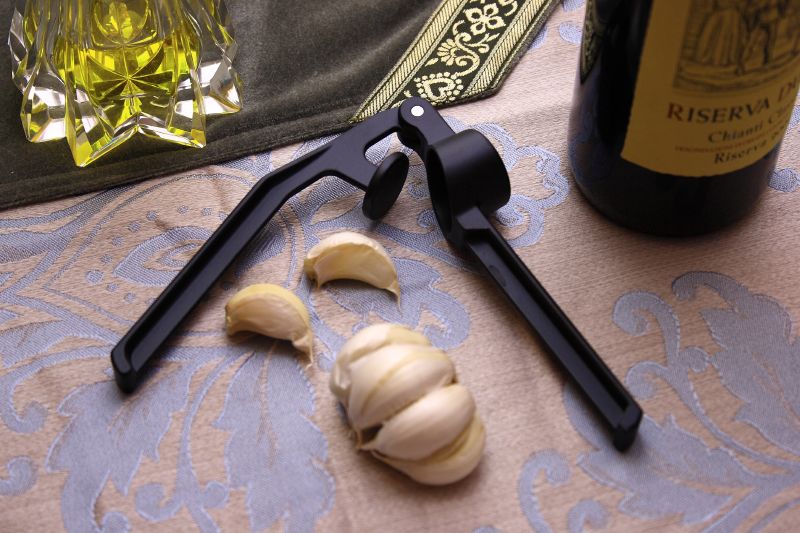This horizontally aligned rectangular picture showcases a beautifully set surface, potentially a table, adorned with a fabric featuring a sophisticated leaf pattern with gray leaves and swirling lines on a brown background. Prominently situated in the upper right-hand corner, an upright wine bottle is partially visible, displaying a brown label inscribed with "Reserva." At its base, a circular nutcracker, equipped with two black handles, holds a few cracked nuts at its center, indicative of recent use. In the upper left-hand corner, a glass vial containing a yellow liquid—likely oil—stands upright, adding a vibrant hue to the scene. Beside it, dark gray cloth underscores the vial’s placement. Overall, the assortment of objects, including the garlic cloves likely mistaken earlier for cracked nuts, nutcracker, wine bottle, and oil bottle, suggests an indoor setting, possibly a cozy kitchen, bar area, or dining hall, illuminated in natural daylight.